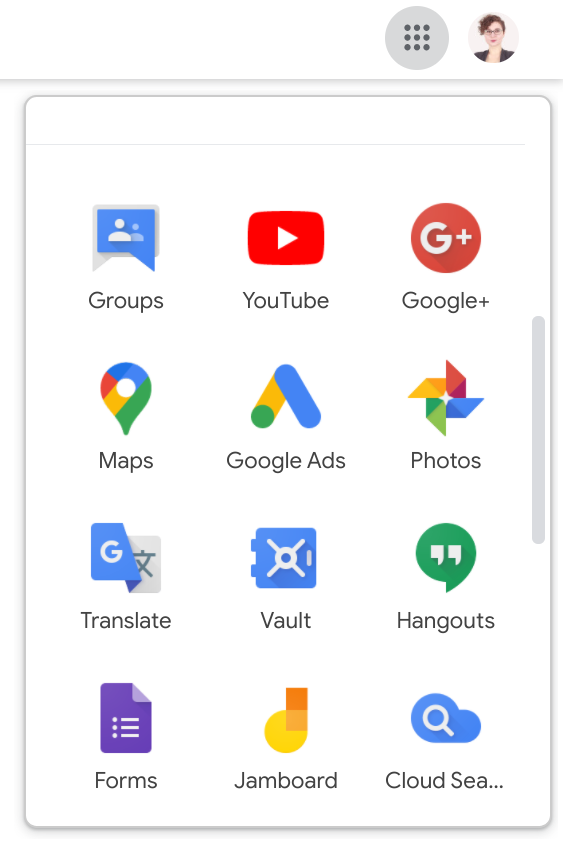The image is a detailed screenshot from a Google interface. In the upper right-hand corner, there is a grid icon comprising nine black circles arranged in three rows and three columns. Adjacent to this icon is an avatar depicting a light-skinned woman with red hair, glasses, and a black jacket. Below this section runs a gray horizontal line that spans the width of the page.

Directly beneath, a pop-up bar appears. On its right side, there's a vertical scroll bar, indicating the content can be navigated up and down the page. The main portion of the screenshot displays a grid of icons, organized into three columns and four rows.

- **First Row:**
  - **Groups:** Corresponding icon.
  - **YouTube:** A red, rounded rectangle resembling a television screen with a white play triangle in the center, labeled "YouTube" beneath it.
  - **Google+:** Corresponding icon.

- **Second Row:**
  - **Maps:** Corresponding icon.
  - **Google Ads:** Corresponding icon.
  - **Photos:** Corresponding icon.

- **Third Row:**
  - **Google Translate:** Corresponding icon.
  - **Google Vault:** Corresponding icon.
  - **Hangouts:** Corresponding icon.

- **Fourth Row:**
  - **Forums:** Corresponding icon.
  - **Jamboard:** Corresponding icon.
  - **Cloud Search:** Corresponding icon.

Each icon represents a Google service, with distinct visuals for easy identification, such as the red YouTube icon with a white play button.